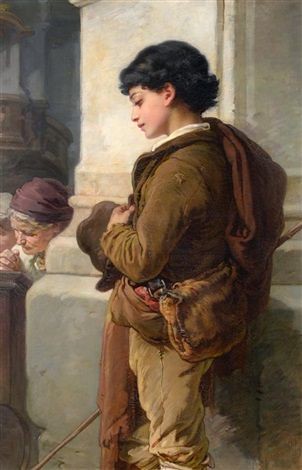This artwork is a detailed painting portraying a solemn young Caucasian boy with dark black hair, dressed in period clothing reminiscent of the early 20th century. He stands prominently in the forefront next to a white marble column. The boy is attired in a brown suede jacket and khaki pants, with a white shirt collar peeking out from underneath. He carries a cross-body satchel draped over his chest, the bag hanging on his left side, and clutches a hat in his left hand. Additionally, he holds a stick in his right hand, partially obscured by his body. A blanket hangs over his right shoulder and a reddish item is tucked into his pocket. In the background by the column, there is a glimpse of an elderly woman with white hair, donning a purplish headdress, who appears to be in a posture of prayer or leaning on a pew. The overall mood of the painting is somber, reflecting a sense of quiet reflection or introspection.